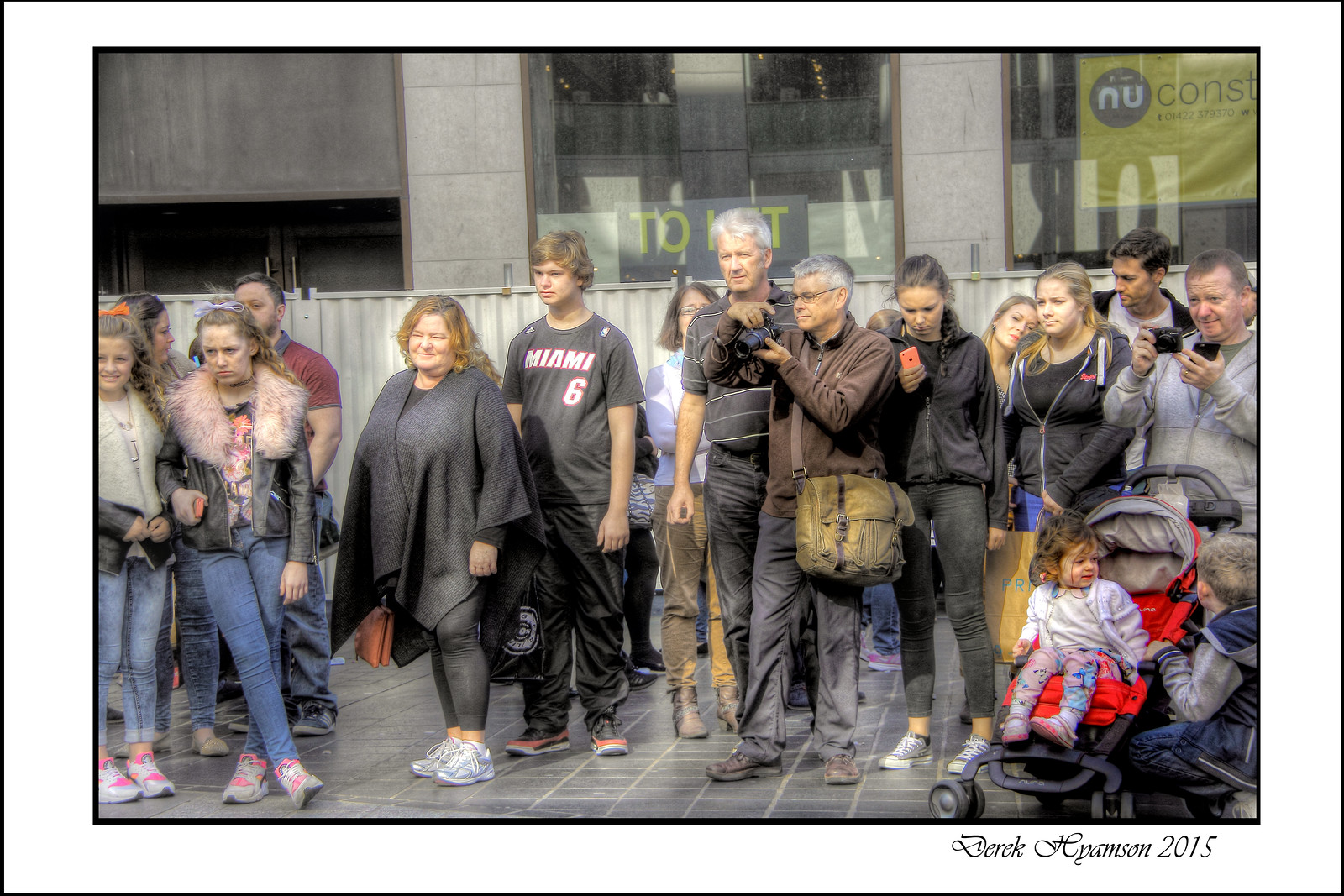A large group of people is posing for a photo outside a gray, metal, or stone building with reflective glass windows, which displays the partially visible signage "N-U-C-O-N-S-T" and a phone number, 014-22-379-370. The tiled ground suggests it could be an upscale outdoor or indoor area. Most individuals are dressed informally, with coats, sweaters, or jackets, and many sporting blue jeans or black leggings. Notably, a young man stands central to the group, wearing a short-sleeved Miami basketball shirt labeled "Miami 6," alongside sweatpants and sneakers. To the left, men in red and gray-striped polo shirts are seen, while a woman in a leather coat with a fur collar is also noticeable. The group includes people holding cameras, some smiling and seemingly engaged in picture-taking. On the far right, a little girl in a stroller gazes at a kneeling little boy beside her. Inscribed in the bottom right corner of the image is the name "Derek Hyamson, 2015."